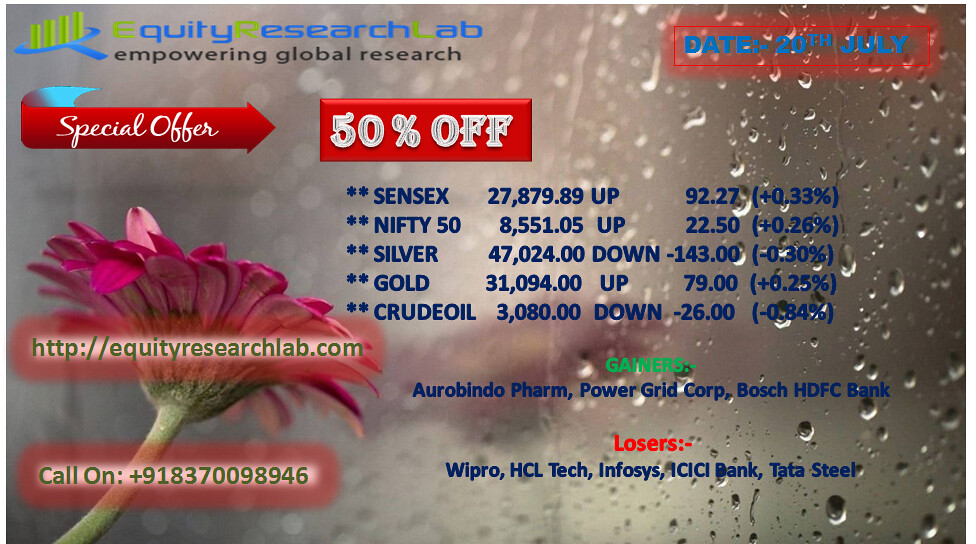This promotional graphic by Equity Research Lab, despite its amateurish design, features a detailed background photo of water droplets on glass with a pink flower and stem on the left. The top of the graphic displays a green and blue logo reading "Equity Research Lab," with "E-R-L" in green, and "Empowering Global Research" underneath in blue. A glowing red-bordered date of "20th of July" is displayed prominently. An arrow indicates a "Special Offer, 50% off," followed by detailed stock information: Sensex at 27,879.89, up by 92.27 points (+0.33%); Nifty 50 at 8,551.05, up by 22.50 points (+0.26%); Silver at 47,024, down by 143 points (-0.30%); Gold at 31,094, up by 79 points (+0.25%); and Crude Oil at 3,080, down by 26 points (-0.84%). The graphic also lists gainers (in green) - Aurobindo Farm, Power Grid Corp, Bosch HDFC Bank - and losers (in red) - Wipro, HCL Tech, Infosys, ICICI Bank, Tata Steel. There is a glowing box over the flower that includes the URL http://equityresearchlab.com, and a phone number: +91 837 009 8946.